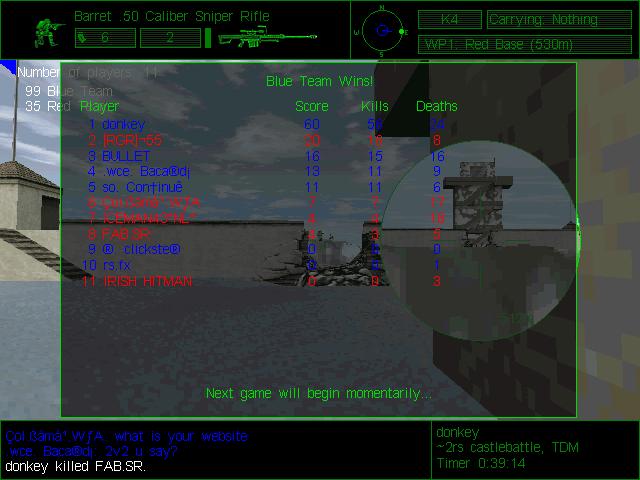This image captures a screenshot from a vintage first-person shooter video game featuring a simplistic user interface with minimal graphic elements. The top and bottom sections of the screen are bordered by black bars. At the top left corner, there's detailed weapon information including a Barrett .50 caliber sniper rifle, shown alongside an illustration of a crouching green army man. Most of the user interface consists of basic, transparent line boxes with sections highlighted in green.

The central gameplay area resembles a war zone with debris or sandbags, partially blown-out buildings, and general battlefield chaos. Player names are displayed in blue and red, indicating team affiliations. The heads-up display (HUD) shows vital game statistics such as scores, number of kills, and deaths. The blue team is indicated as the winner with a message in lime green text stating that the next game will begin momentarily. 

Additionally, there is a circular mini-map or compass on the screen to help players with navigation. At the bottom of the screen, specific in-game events are shown, including "donkey killed fab.sr," with further details indicating "donkey, castle battle, timer 3914." The overall feel of the interface is utilitarian, reminiscent of early PvP shooter games with a clear and functional design focus.